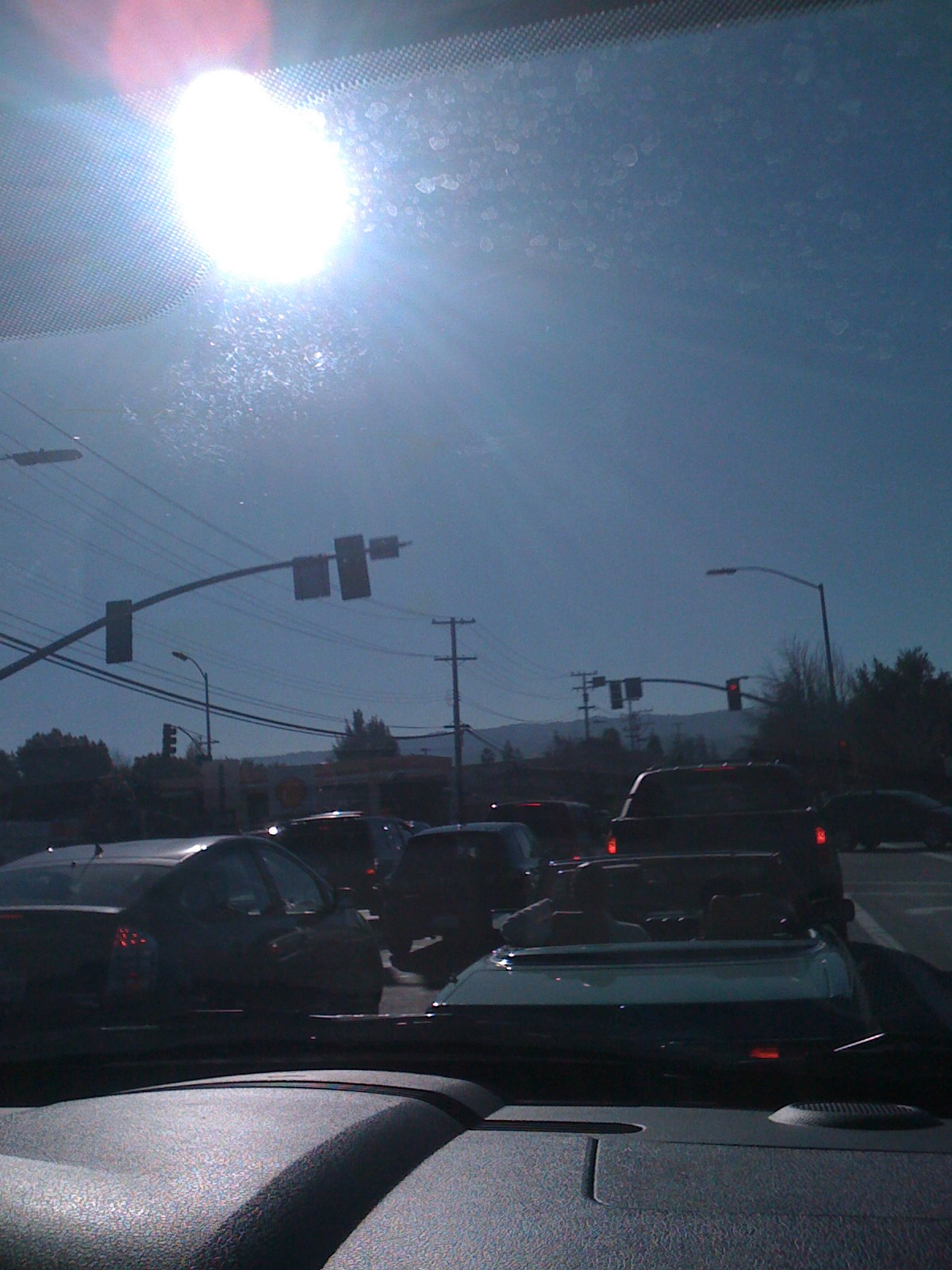This detailed daytime photo captures a traffic stop scene from inside a car, viewed from the dashboard, which is notable for its grey-black color. The windshield reveals dirt smudges and water spots, reflecting the bright sun located in the top left corner of the image, its rays faintly visible. The sky is a clear blue, and distant trees add to the setting. Ahead, the traffic light glows red, halting vehicles in their tracks. Directly in front of the photographer's car, which is in the right lane, there are approximately two to three cars, including a distinctive teal convertible. To the left, several more vehicles wait. The left side of the image also shows traffic signals, city lights, electrical wires, and a Shell gas station.